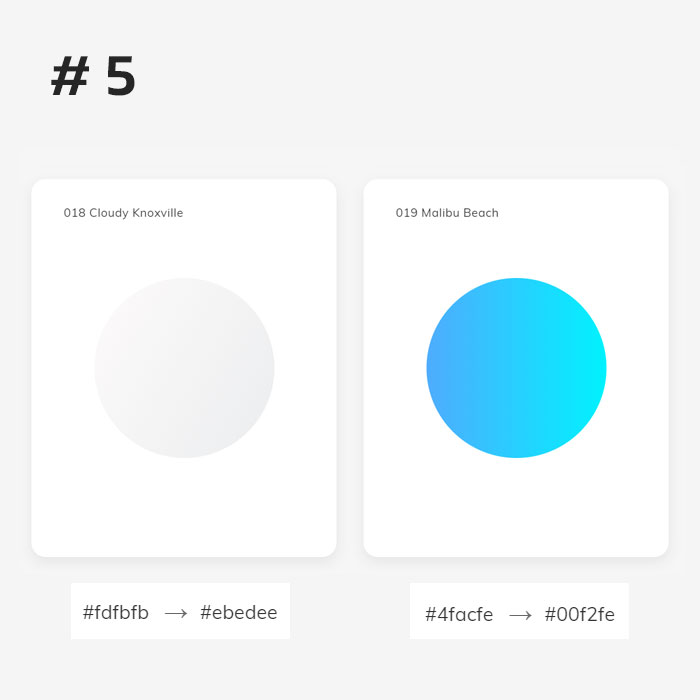This image features a visually striking composition with vibrant color elements set against a gray background. Prominently displayed in the top left corner is a large black numeral "5". 

Near the top of the image, there are two substantial white squares with colored circles at their centers. The left square is titled "018 Cloudy Knoxville," showcasing a circle filled with a grayish-white hue. Directly beneath the circle is a white rectangle containing the color codes: "#FDFBFB" flanked by an arrow pointing right to "#EBEDEE".

Adjacent to it on the right, the other square is labeled "019 Malibu Beach," illustrating a gradient blue circle that transitions from a darker blue on the left to a lighter blue on the right. Below this gradient, a white rectangle presents the corresponding color codes: "#4FACFE" pointing right to "#00F2FE".

The meticulous layout and specific color details provide a clear and organized presentation of these two color schemes.